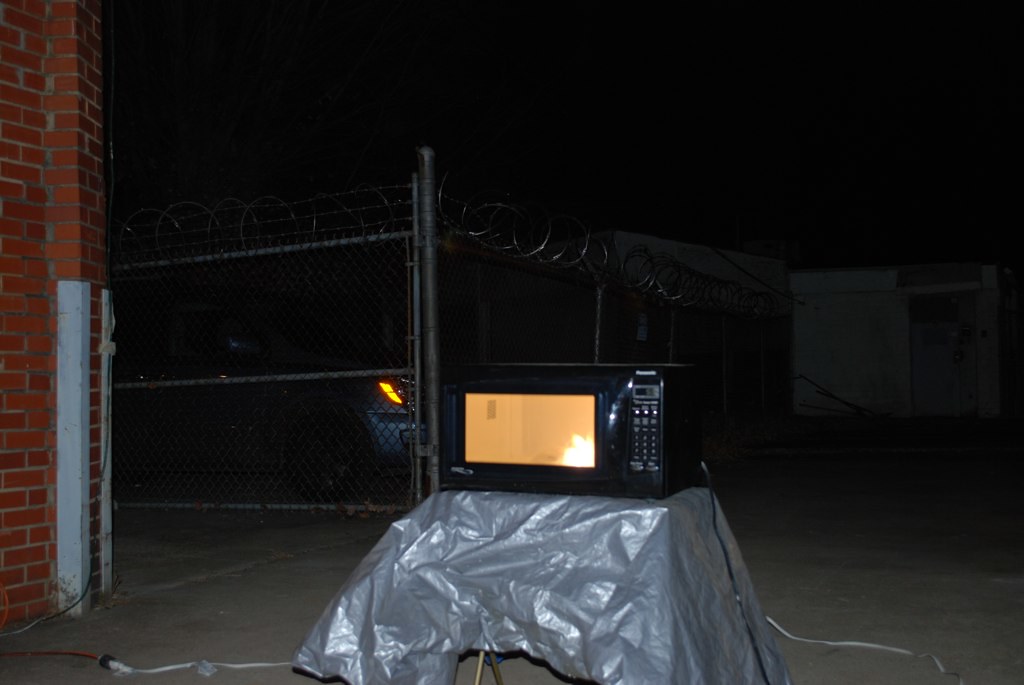This striking nighttime photograph captures an outdoor scene reminiscent of the YouTube show "Is it a Good Idea to Microwave This?". Centered on a small, black microwave that appears to be intensely microwaving something to the point of catching fire, the image radiates a sense of controlled chaos. The microwave sits on a table, which is covered with a grayish-silver tarp, likely as a safety measure to prevent the fire from spreading. The scene is set against a backdrop of a chain-link fence adorned with wires at the top and accompanied by parked cars and a brick wall on the left side. The ground is paved with concrete, adorned with power cables that snake towards the microwave. Light from the burning object inside the microwave reflects off its glass door, despite the appearance of the outer buttons remaining black and undisturbed. This vivid, well-lit spectacle likely aims to test the limits of the microwave under carefully managed conditions.